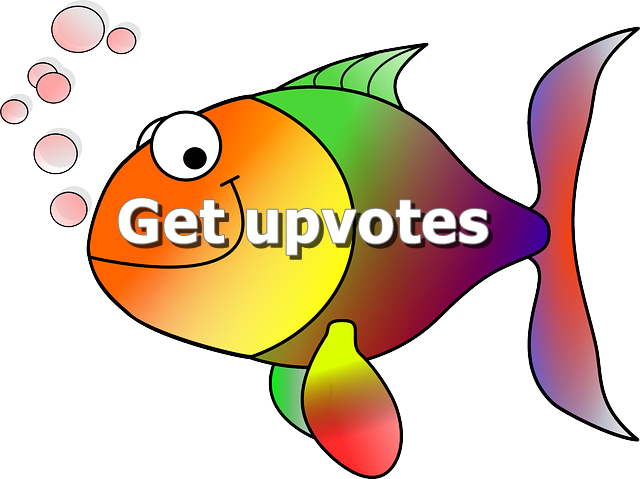The image is a colorful, cartoon-style fish on a white background, facing left. The fish has a round, almond-shaped body with a gradient face transitioning from orange to yellow, adorned with large, white eyes and a big, cartoonish smile. Its body exhibits a vivid gradient from green to reddish-purple. The fish's top fin, which resembles a shark’s fin, is green, while its tail fin blends purple and red. It has two middle fins at the bottom; the front fin shows a gradient from yellow to red, and the partially hidden rear fin is green. Light pink bubbles of varying sizes emerge from the fish’s mouth. Overlaid on the fish's body in white text with a subtle black shadow are the words "get upvotes."